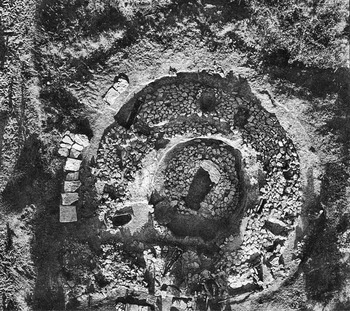The image is a black and white aerial or satellite view depicting a rocky terrain where elevated points cast dark shadows to their south. Central to the image are two concentric circular areas comprised of white rocky ground interspersed with larger dark stones. These circular areas suggest an archaeological site, possibly the remnants of an ancient structure or excavation. Scattered throughout the terrain are various gaps and holes, indicating active or previous digs. In the upper left-hand corner, just outside the second, larger circular enclosure, is a small row of nearly square shapes, possibly rocks or square outbuildings. Additionally, the image features a mix of small gravel and sand, contributing to the rugged texture of the terrain. Overall, the scene appears to be historical ruins viewed from above, with an intricate layout of natural and possibly man-made formations.